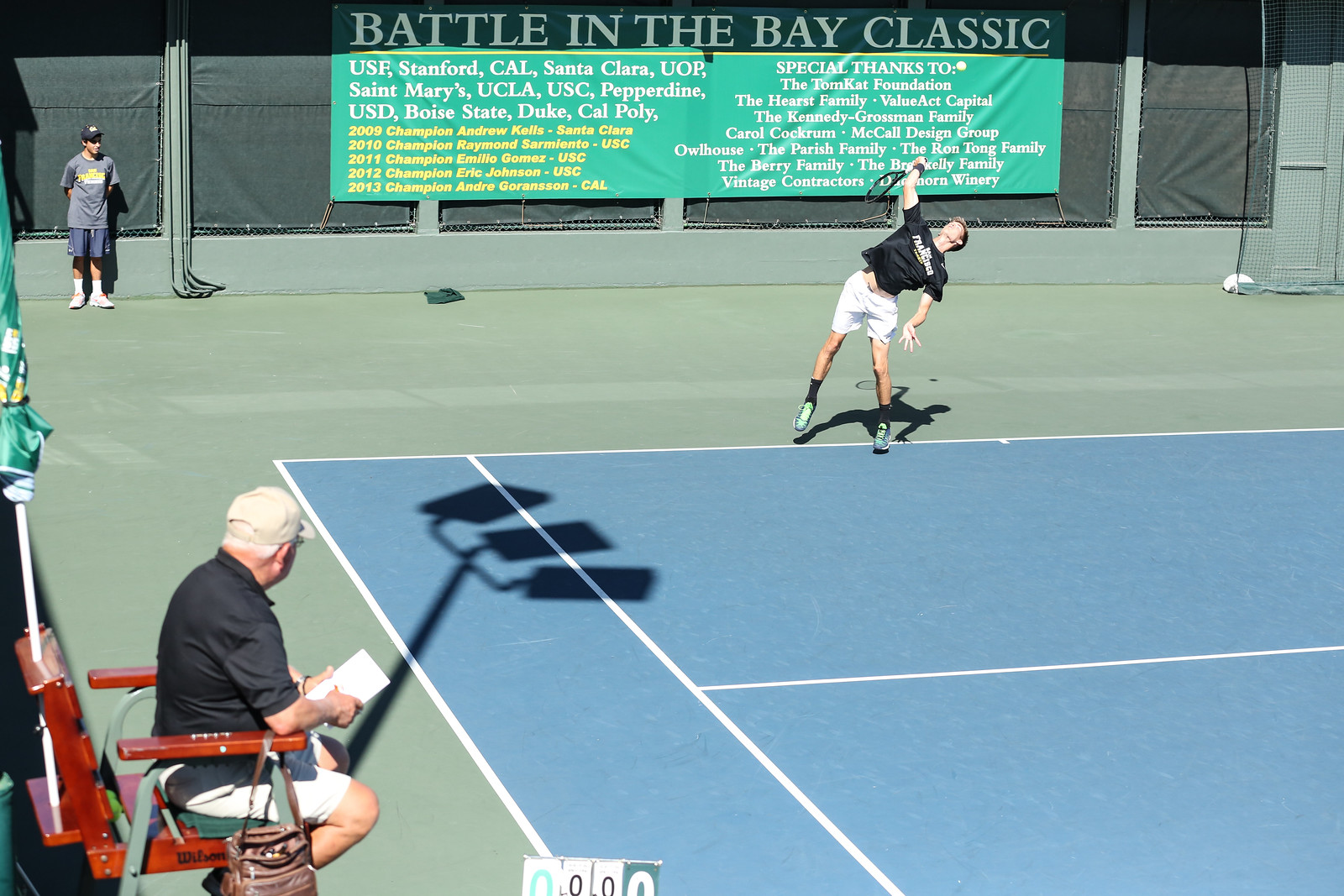In this detailed image of a tennis court during the Battle in the Bay Classic, the focal point is a blue hard court with white lines, bordered by a green perimeter. Positioned at the far end of the court, a young man is captured in mid-serve, dressed in a black shirt and white shorts, facing the viewer. To the left side of the picture, an older man is seated in a wooden fold-out chair, with a purse hanging from the chair's right arm. He dons a black shirt, white shorts, and a white baseball cap, and appears to be observing the match, possibly taking notes as he holds some papers. Additionally, a man in a gray t-shirt, blue shorts, white socks, shoes, and a blue cap stands to the left of the chair. Further back, another figure, likely a ball boy, stands with his hands behind his back.

In the background, a prominent banner reads "Battle in the Bay Classic," listing various participating schools including USF, Stanford, Cal, Santa Clara, Boise State, Duke, Cal Poly, and others, alongside special thanks to sponsors and donors. The photograph, taken in daylight, also shows shadows cast by overhead lights, adding depth to the scene.